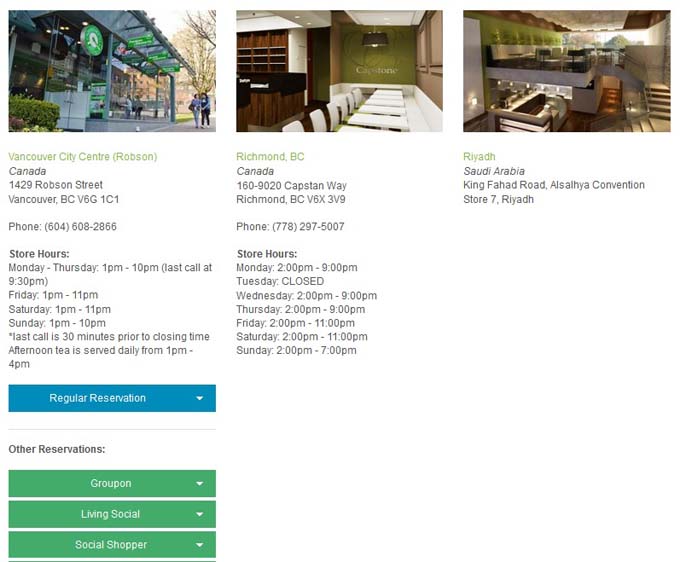Here is a detailed and cleaned-up caption for the described image:

---

This screenshot appears to be taken from a directory page, possibly related to reservations. The cropped image features three distinct sections, each displaying different images along with informative text beneath them.

1. The first section showcases an image of what seems to be the exterior of a shopping area, closely resembling a coffee shop or café. The accompanying text reads:
   - **Vancouver City Centre (Robson), Canada**
   - **Address:** 1429 Robson Street, Vancouver, BC, V6G 1C1
   - **Phone Number:** 604-508-2866 or 604-508-2856
   - **Store Hours:**
     - Monday to Thursday: 1 PM - 10 PM (Last call at 9:30 PM)
     - Friday and Saturday: 1 PM - 11 PM
     - Sunday: 1 PM - 10 PM (Last call 30 minutes before closing)
   - **Additional Information:** Afternoon tea is served daily from 1 PM to 4 PM.
   - **Reservation Options:** 
     - A blue button labeled "Regular Reservation" that includes a dropdown menu.
     - Three green buttons for different group reservations labeled "Groupon," "Living Social," and "Social Shopper."

2. The second section features an image resembling a hotel dining room, potentially a breakfast area typical of a continental breakfast setup:
   - **Richmond, BC, Canada**
   - **Location:** Capston Way, Richmond, BC
   - **Store Hours:**
     - Monday, Wednesday, Thursday: 2 PM - 9 PM
     - Tuesday: Closed
     - Friday and Saturday: 2 PM - 11 PM
     - Sunday: 2 PM - 7 PM
   - **Note:** This section does not provide reservation buttons or options.

3. The third section presents an image of a modern indoor space, identified as:
   - **Riyadh, Saudi Arabia**
   - **Address:** King Fahad Road, Convention Store 7, Riyadh
   - **Note:** No store hours or reservation options are provided for this location.

---

This descriptive caption provides a clear and comprehensive summary of the contents depicted in the screenshot.